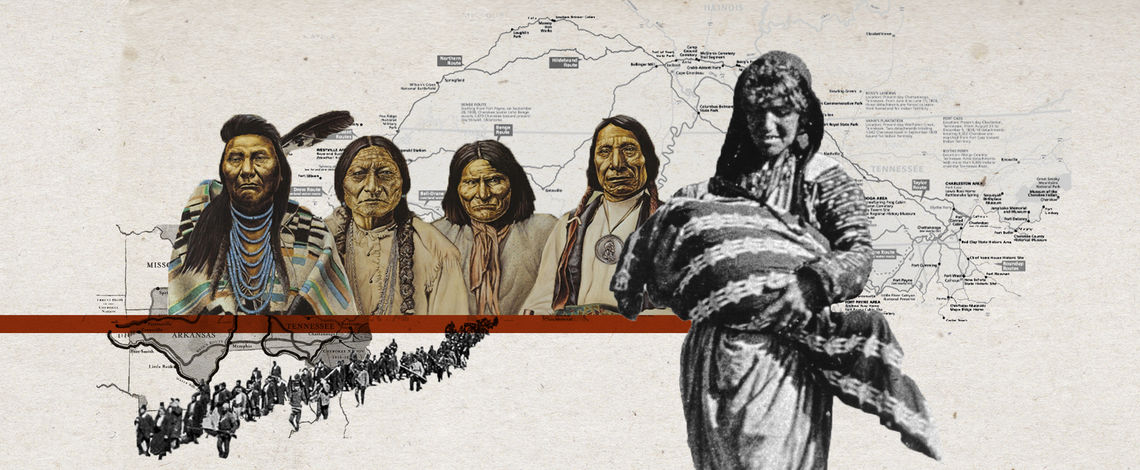The image appears to be an intricate historical illustration, possibly from a history book, depicting five Native Americans against a backdrop of a black and white map showing various geographies, including Arkansas, Missouri, and Tennessee, though the map's details are too small to decipher clearly. Four of the individuals, presumably men, are vividly colored and drawn, while the fifth figure, a woman on the far right, is represented by an imposed black and white photograph. The woman, seemingly holding a baby wrapped in a blanket and adorned in various robes, stands out prominently. 

The illustration suggests a timeline or scene along the Trail of Tears, with visual elements evoking a somber journey; a thick red line runs through the middle of the depicted Native Americans, perhaps symbolizing the path or divide of this historical event. Notably, one Native American man wearing a feathered headdress and beaded necklace appears to be a chief, his dignified stance contrasting with the relatively simpler attire of the other men. Emotional expressions vary among the individuals: the chief and woman appear content, while the remaining three men display anger or sternness.

Beneath the central figures, the map extends to show a large group of Native Americans walking in a line, further emphasizing the massive displacement associated with the Trail of Tears. All these elements combined create a detailed and poignant portrayal of a significant period in Native American history.